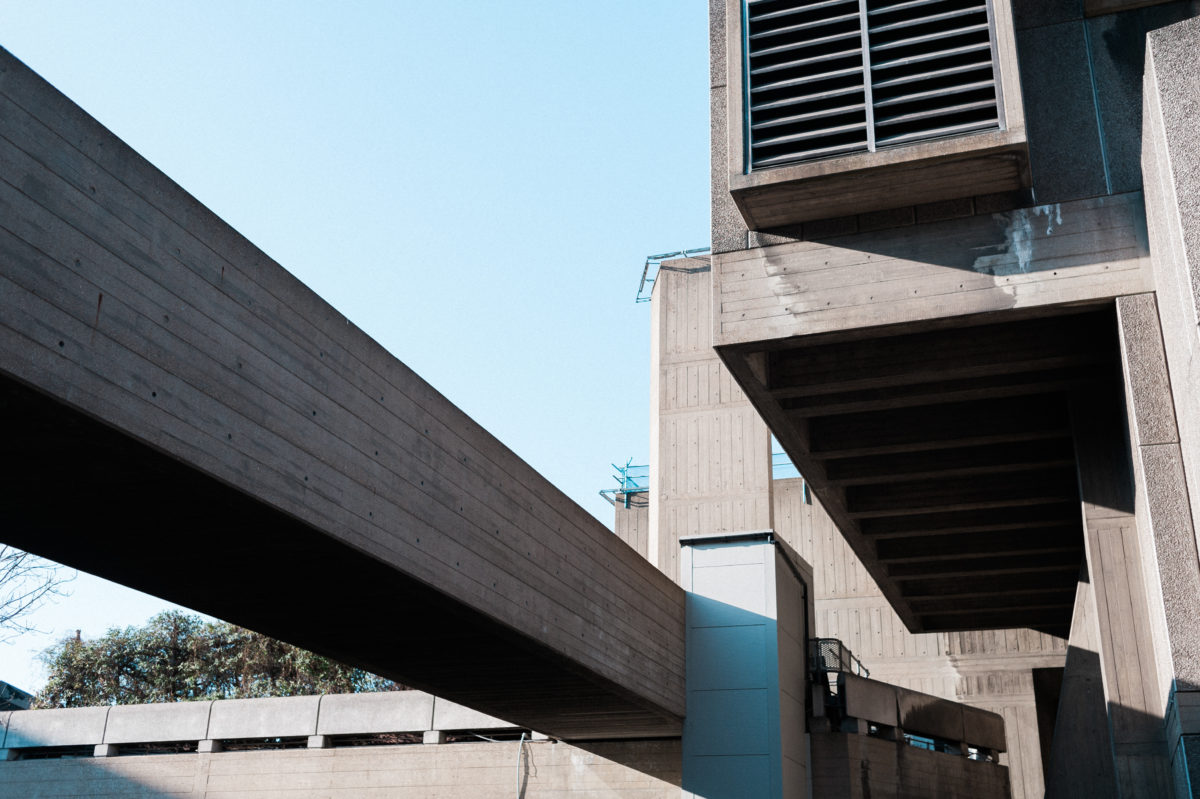The image depicts an old, industrial-looking gray building under construction, featuring a noticeable vent or grate near the top. The building, characterized by its blocky, concrete appearance and dark shadowing, has streaks of what might be white paint or mold. A large beam, possibly wooden but potentially metal, extends prominently from its side. Situated predominantly on the right side of the photo, the structure contrasts with a backdrop of light blue sky and surrounding trees. The photograph, taken during the daytime, highlights the varying shades of gray and black on the building, with the shadows providing depth and indicating different angles and portions of the construction.